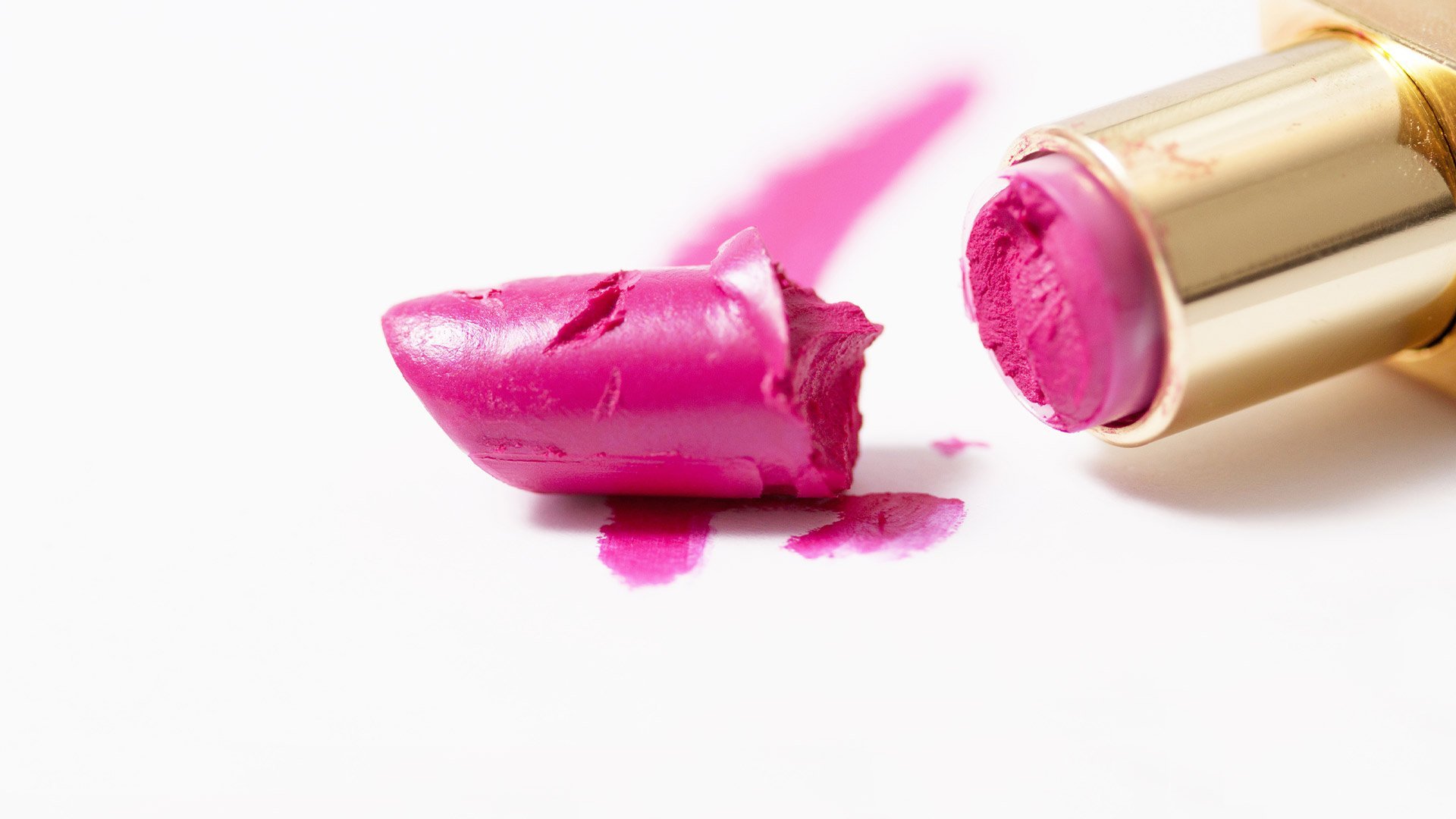The image showcases a broken pink lipstick tube on a white background. The lipstick has cleanly snapped off at the tip, leaving the broken piece lying separately on the white surface, creating a noticeable pink smear below it. The remaining part of the lipstick, housed in a gold tube, is visible, although the cap is missing. The severed piece of lipstick appears to have bite marks or scratches, adding a distressed look, and its smooth, slightly curved surface resembles a decapitated finger's tip. Additionally, there are light scratching and ridges around the area where it broke, making the damage look severe. The overall condition of the lipstick suggests it has not been used much and the gold tube appears square with a round base housing the remaining lipstick. The pink shade also has subtle blue highlights, enhancing its color.